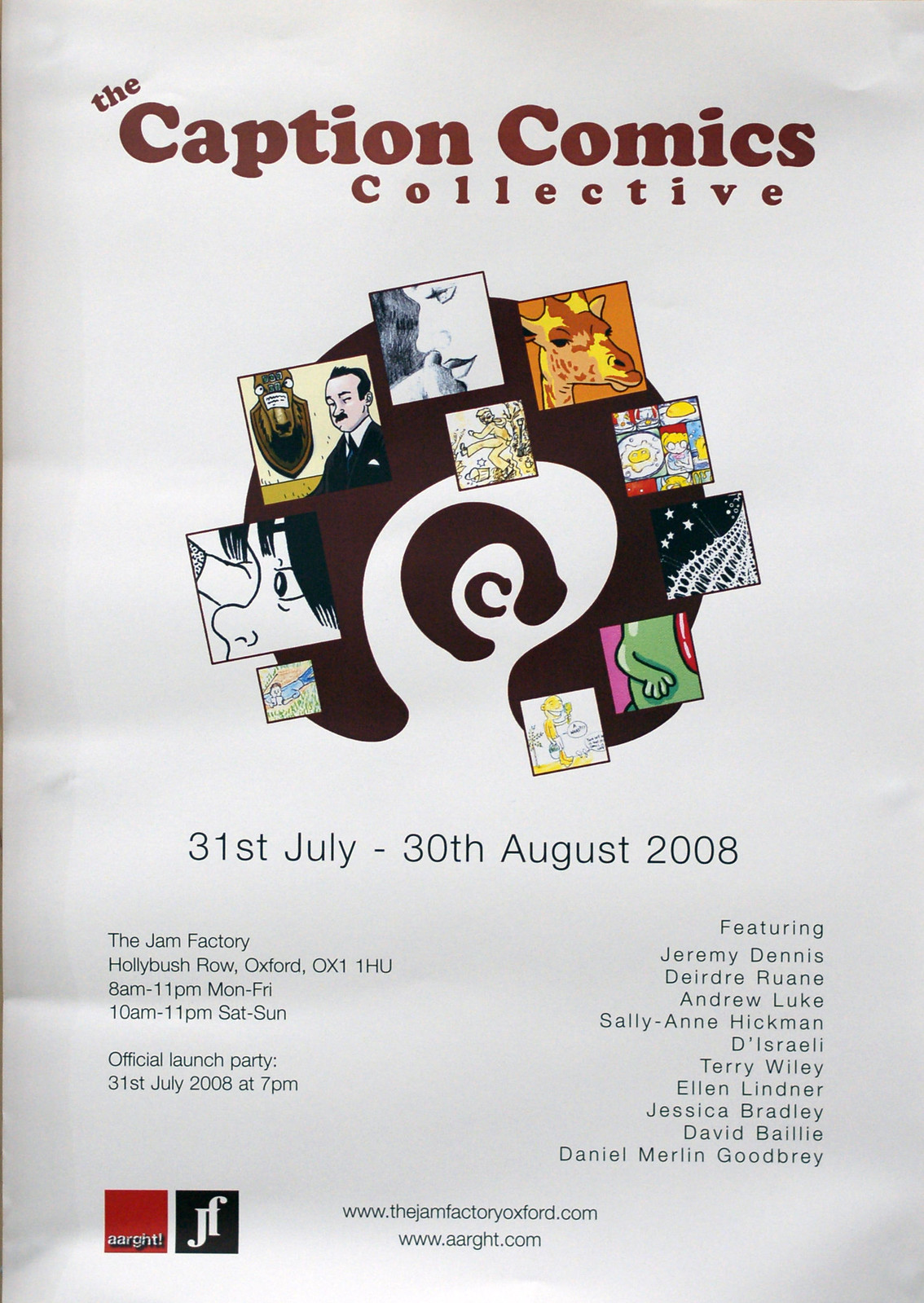This vibrant poster for the Caption Comics Collective features a prominent header in brown text, displaying the group's name. Below, an array of about ten varied artworks encircles an abstract illustration set against a captivating black swirl. The artworks include detailed images such as a giraffe, a man's face, and pieces of more abstract art, each contributing to the eclectic visual display.

The event details span the bottom half of the poster, announcing the exhibition dates from 31st July to 30th August 2008, held at The Jam Factory, Hollybush Row, Oxford, OX1 1HU. The venue hours are listed as 8 a.m. to 11 p.m. from Monday through Friday, and 10 a.m. to 11 p.m. on weekends. An official launch party is highlighted for 31st July 2008 at 7 p.m.

The poster also prominently features the names of participants including Jeremy Dennis, DeAndre Ron, Andrew Luke, Sally Ann Hickman, Dee Israeli, Terry Wiley, Ellen Lindner, Jessica Bradley, David Bally, and Daniel Merlin Goodbray. At the bottom left corner are two logos: a simple red box and a 'JF' in red. The poster also provides a link to further details at www.thejamfactoryoxford.com.